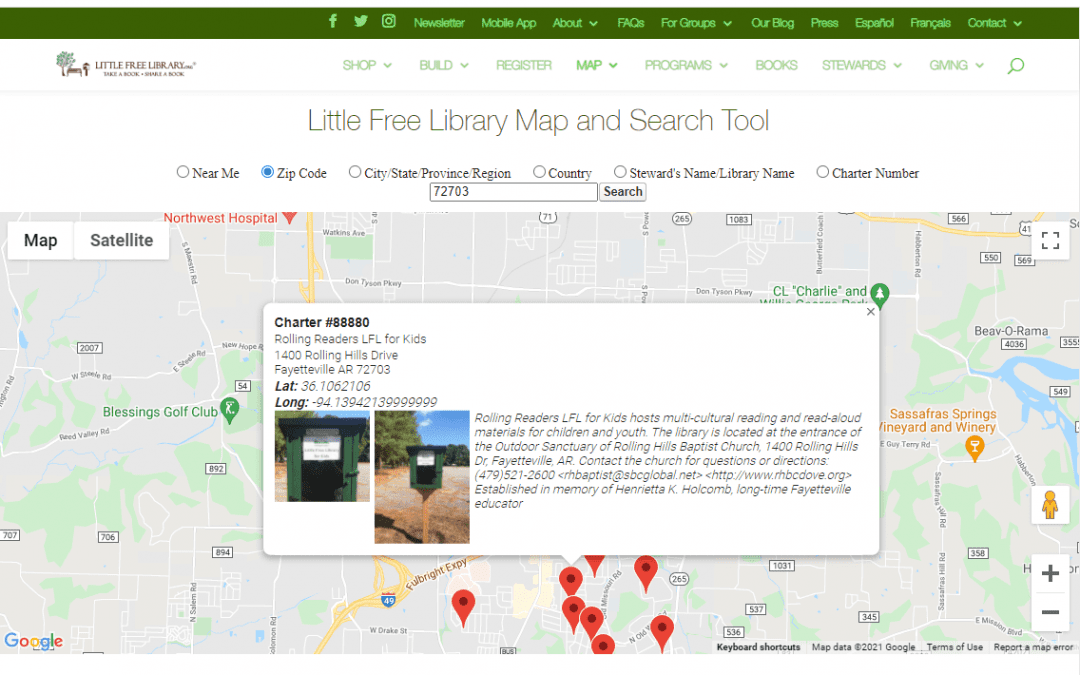A detailed visual description of the screenshot:

The screenshot predominantly features a section of Google Maps, characterized by various colors and text elements:

- **Top Section**: 
  - The uppermost area is a green bar with bold white text.
  - Below the green bar, there is a white strip displaying black text.

- **Main Body**: 
  - The main section of the screenshot is a Google Maps interface.
  - In the top left corner, there's a "Map" and "Satellite" toggle option housed in a white rectangular background.
  - Multiple red location markers/bubbles are scattered across the map.

- **Overlay and Markers**:
  - Overlaid on the map, there is a white box with the title "Charters" in black letters, followed by some illegible numbers.
  - Two photos of a green box on a yellow post are visible; the green box features a white sign at its center.

- **Interactive Elements**:
  - The bottom right corner has plus and minus symbols within white squares for zooming in and out.
  - Above these symbols, there's a yellow icon inside a white square, resembling a "penis" symbol.
  - The bottom left corner displays the word "Google" as part of the Google Maps watermark.
  - In the top right corner of the map, there's a fullscreen button enclosed in a white square.

Each element contributes to a detailed presentation of a Google Maps interface, overlaid with specific markers, photos, and interactive icons.